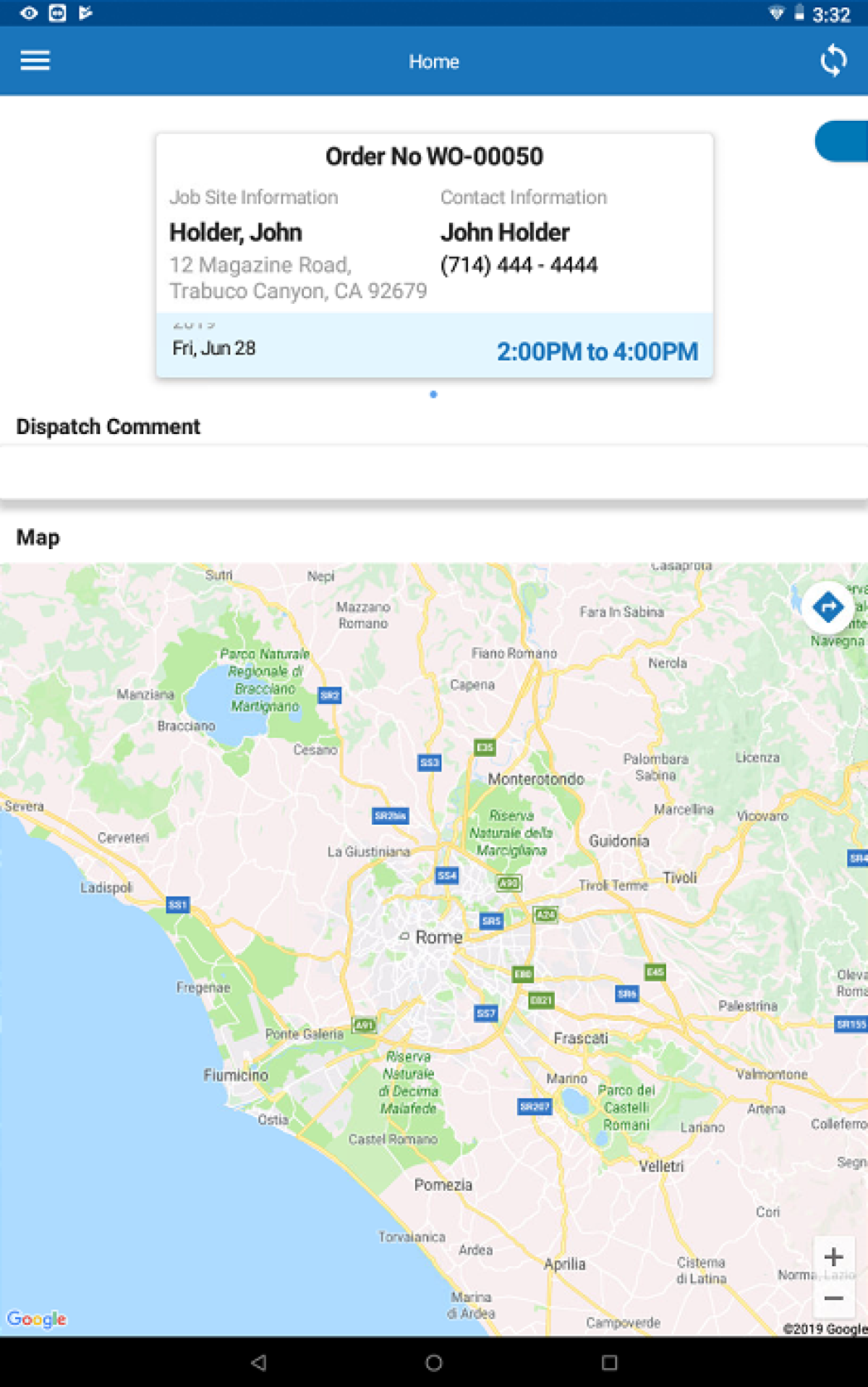This image is a screenshot captured from a smart device, likely a mobile phone or tablet. At the top of the screen, there are status icons commonly found on such devices, including indicators for Wi-Fi connection, battery level, and the current time. The screenshot displays the interface of a mobile application, characterized by a blue rectangular bar at the top. On this bar, there are three white vertical lines in the top left corner, a circular arrow icon in the top right corner, and the word "HOME" centered in the middle.

The main content of the screenshot details an order, featuring an order number, contact information including a name and phone number, a delivery address designated for a job site, and a scheduled date and time for the delivery: Friday, June 28th, from 2 pm to 4 pm. At the bottom of the image, there is a map provided by Google Maps, specifically highlighting the city of Rome, the capital of Italy.